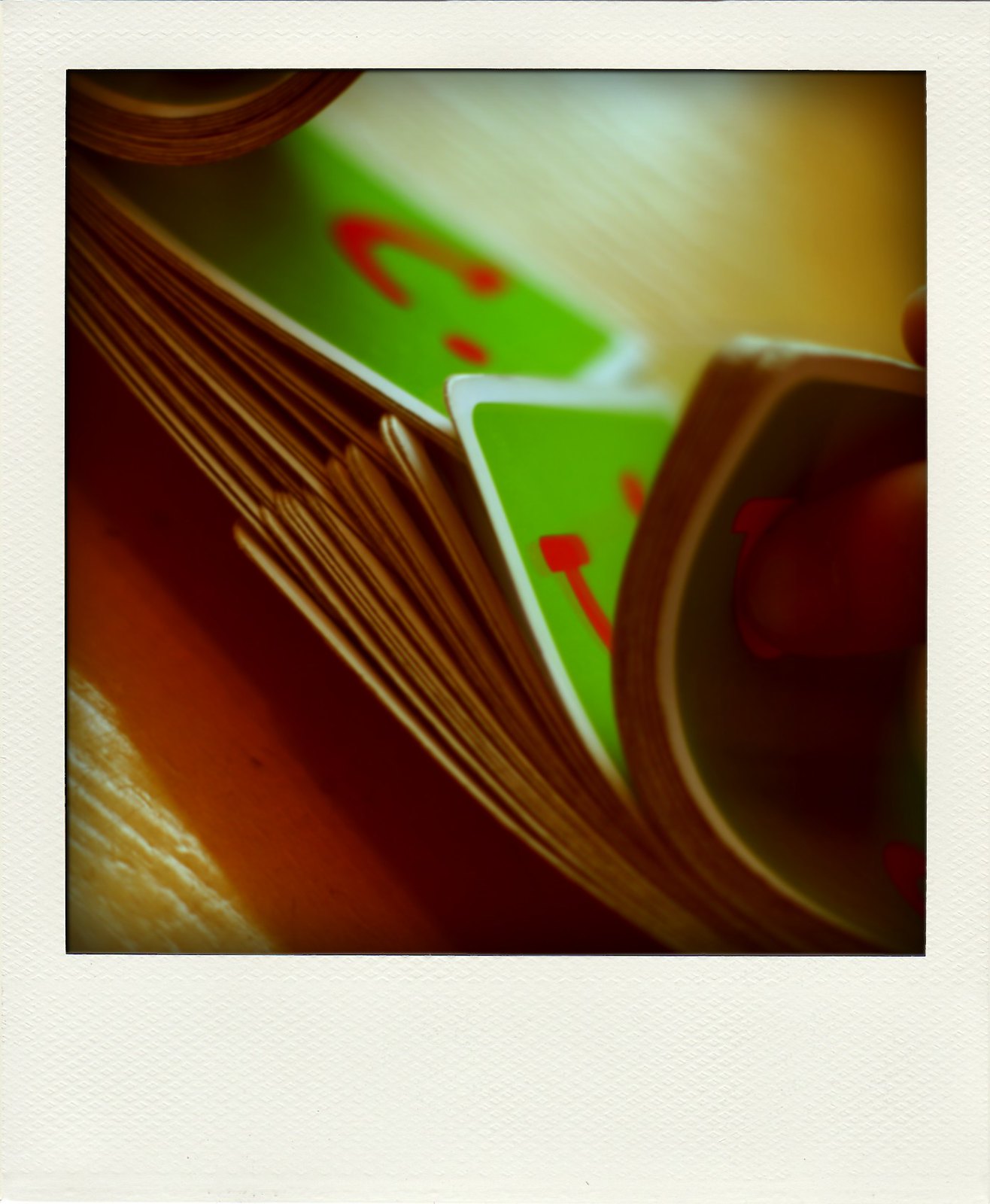In this photograph, a deck of playing cards is being skillfully bridge shuffled together. The image captures the precise moment when the two halves of the deck are pushed into each other, creating a dynamic arch in the center as the cards intermingle. On the right-hand side of the photo, a pair of fingers is visible, applying pressure to facilitate the shuffle process, demonstrating the physical dexterity required for this technique. The card backs sport a unique design featuring a greenish background bordered with white, and a distinctive red symbol resembling a U-shape with a dot above it. The action takes place on a grainy-textured tabletop, suggesting a rough playing surface. While the shuffle technique is typically associated with poker cards, the specific type of cards remains unidentified as only the backs are visible. The intricate shuffling method, performed swiftly and efficiently, ensures a thorough and even randomization of the cards, an essential aspect of card games to maintain fairness and unpredictability.